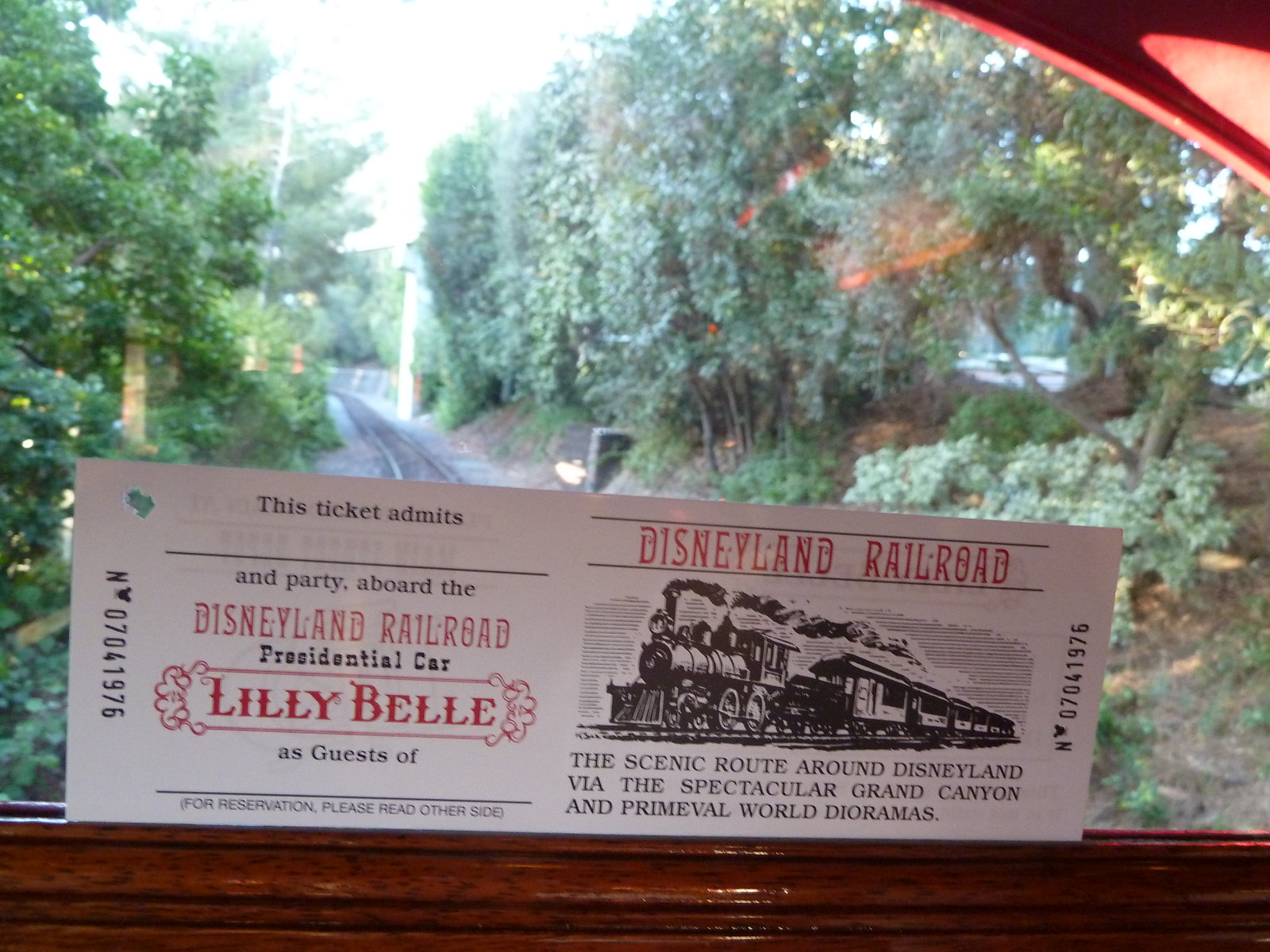The photograph captures a view from inside a railway car, looking out through a window at a scene dominated by tall trees lining either side of visible train tracks. The sky appears overcast, casting a white backdrop over the scene. Affixed horizontally in the groove of the dark, shiny wooden window ledge is a white ticket for the Disneyland Railroad. The ticket's text includes "This ticket admits" followed by a blank space and then "and party aboard the Disneyland Railroad Presidential Car, Lily Bell." "Lily Bell" is emphasized in bold red letters, accompanied by a decorative floral design. On the right side of the ticket, also in red print, it says "Disneyland Railroad," beside a black and white sketch of a steam engine train. Below the image, it reads, "The scenic route around Disneyland via the spectacular Grand Canyon and primeval World Dioramas." This image blends a nostalgic railway journey with a whimsical Disneyland experience.